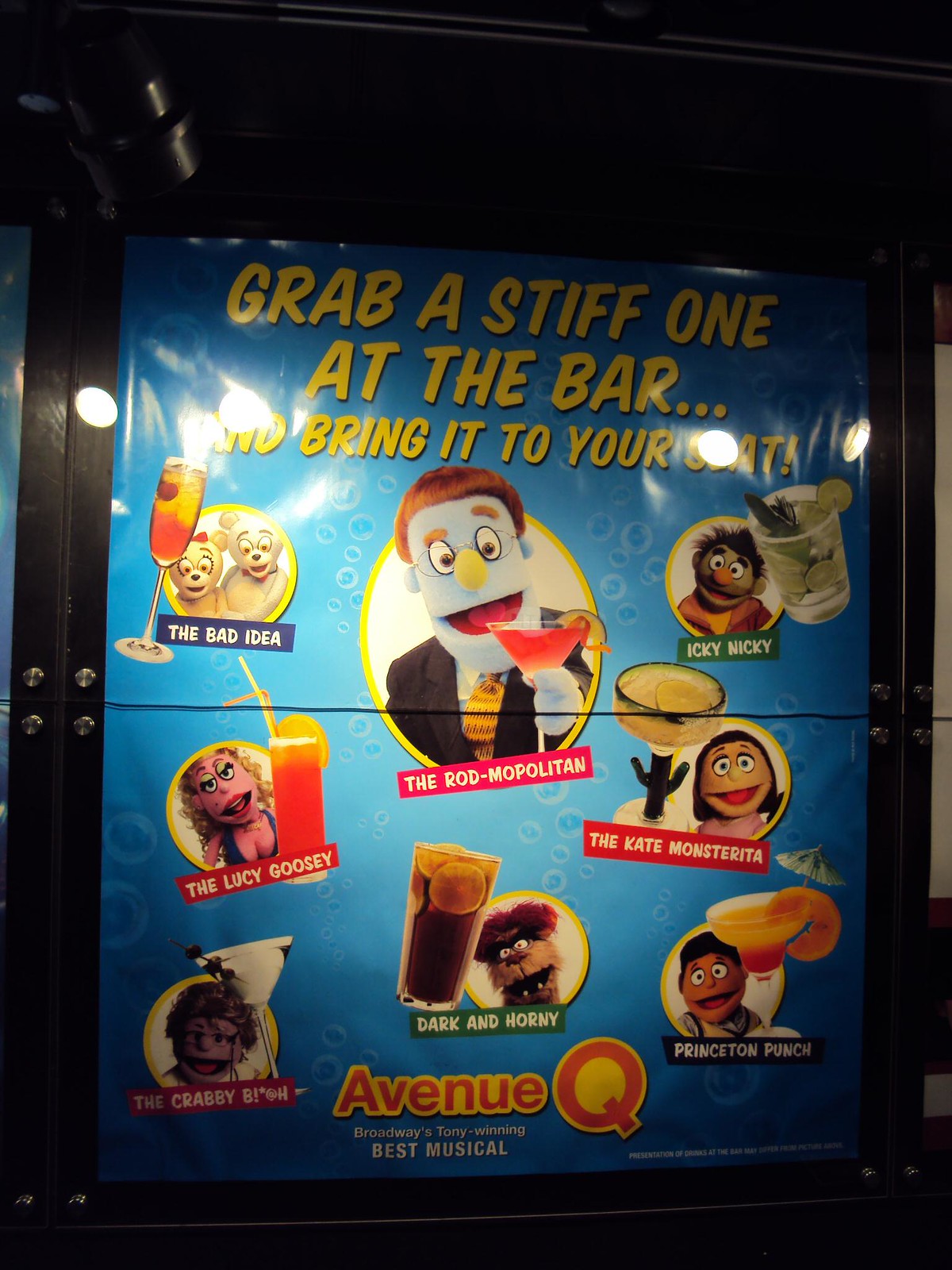The image showcases a detailed poster for the Broadway show Avenue Q. The poster possesses a blue background with underwater bubbles and is displayed behind a clear plastic window. Dominating the top section, in bold yellow text, it reads: "Grab a stiff one at the bar and bring it to your seat." This phrase is partially obscured by glare. 

Centered on the poster, a prominent blue puppet with red hair, reminiscent of Conan O'Brien, is depicted holding an orange margarita. Surrounding this central figure are various smaller circular thumbnails of different puppets, each advertising a unique cocktail. 

Starting from the top left, the puppets and their corresponding drinks are as follows: two teddy bear-like puppets labeled "Bad Idea," a puppet resembling a woman with cleavage for the "Lucy Goosey" cocktail, and an elderly-looking puppet with reading glasses called the "Crabby Bitch." The center of the poster highlights the blue puppet promoting the "Rod Mapolitan." Below this, a puppet that visually mimics Oscar the Grouch but features brown fur and wild reddish hair is labeled "Dark and Horny."

On the right side, positioned at the top, is a puppet endorsing the "Icky Nicky" cocktail. Further down, another puppet presents the "Kate Monsterita," and finally, at the bottom right, the "Princeton Punch" is advertised. At the very bottom of the poster is the logo for Avenue Q, proudly noting it as Broadway's Tony-winning Best Musical.